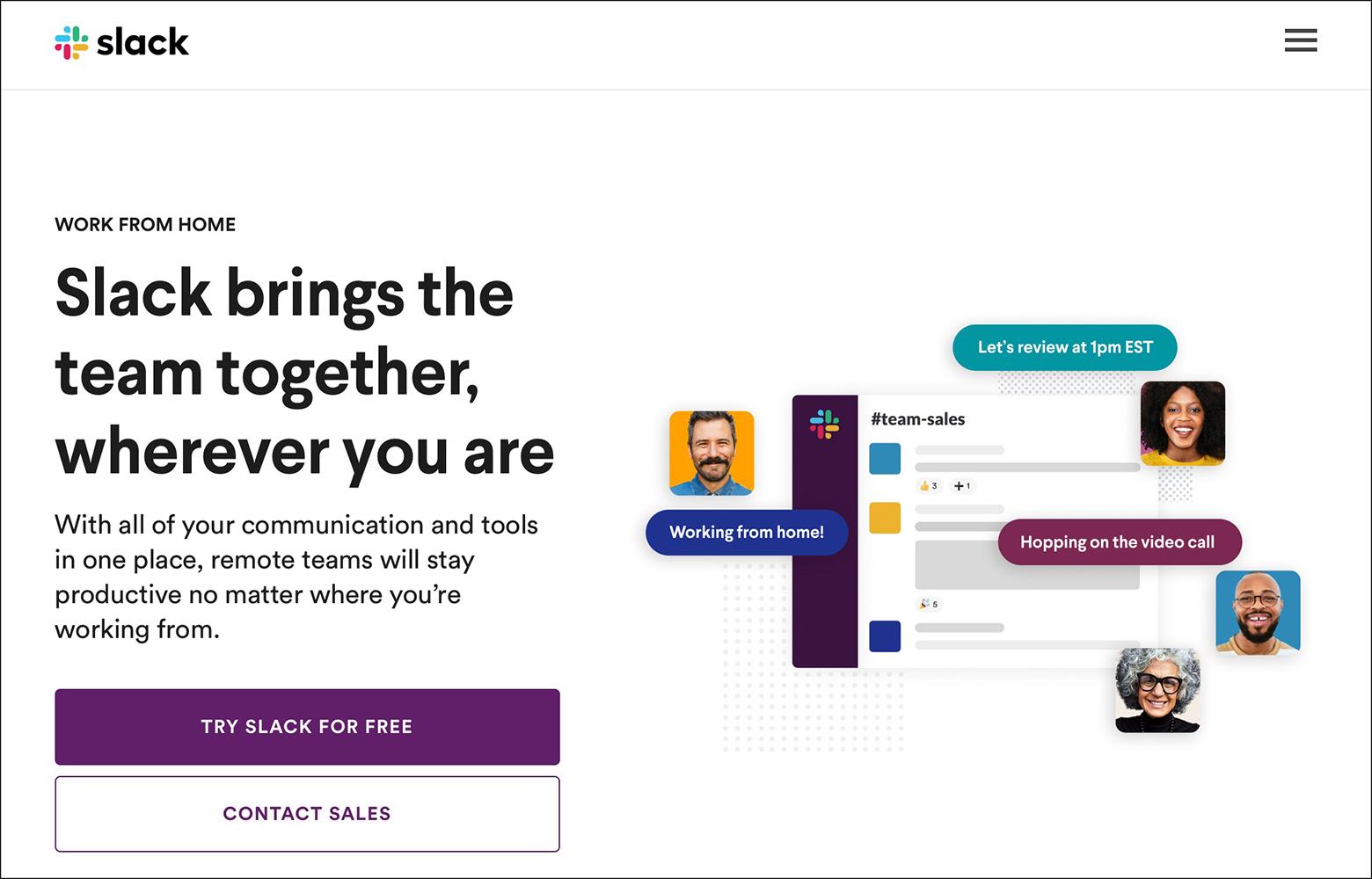The website homepage of Slack is prominently showcased with its recognizable logo at the top—comprising turquoise, green, red, and yellow colors. On the top right, there are three horizontal lines indicating a menu for additional options. 

The headline on the homepage reads, "Work from home: Slack brings the team together wherever you are," underscoring its emphasis on remote collaboration. Beneath this, a subheading elaborates, "With all of our communication and tools in one place, remote teams will stay productive no matter where you're working from."

Directly below the text, there are two buttons: a prominent purple one labeled "Try Slack for free" and a white one labeled "Contact Sales," providing visitors immediate options to either start a free trial or reach out for further inquiries.

To the right of these elements, there's a visual illustration. It features a man and a woman engaging in a video conference, with the text "Work from home" and further details about a review scheduled for 1 PM Eastern Standard Time. Additionally, there is an older woman depicted, though she appears not to be speaking in the image.

Overall, the Slack homepage succinctly conveys its value proposition for remote work, with clear calls-to-action and visual elements that support its narrative.